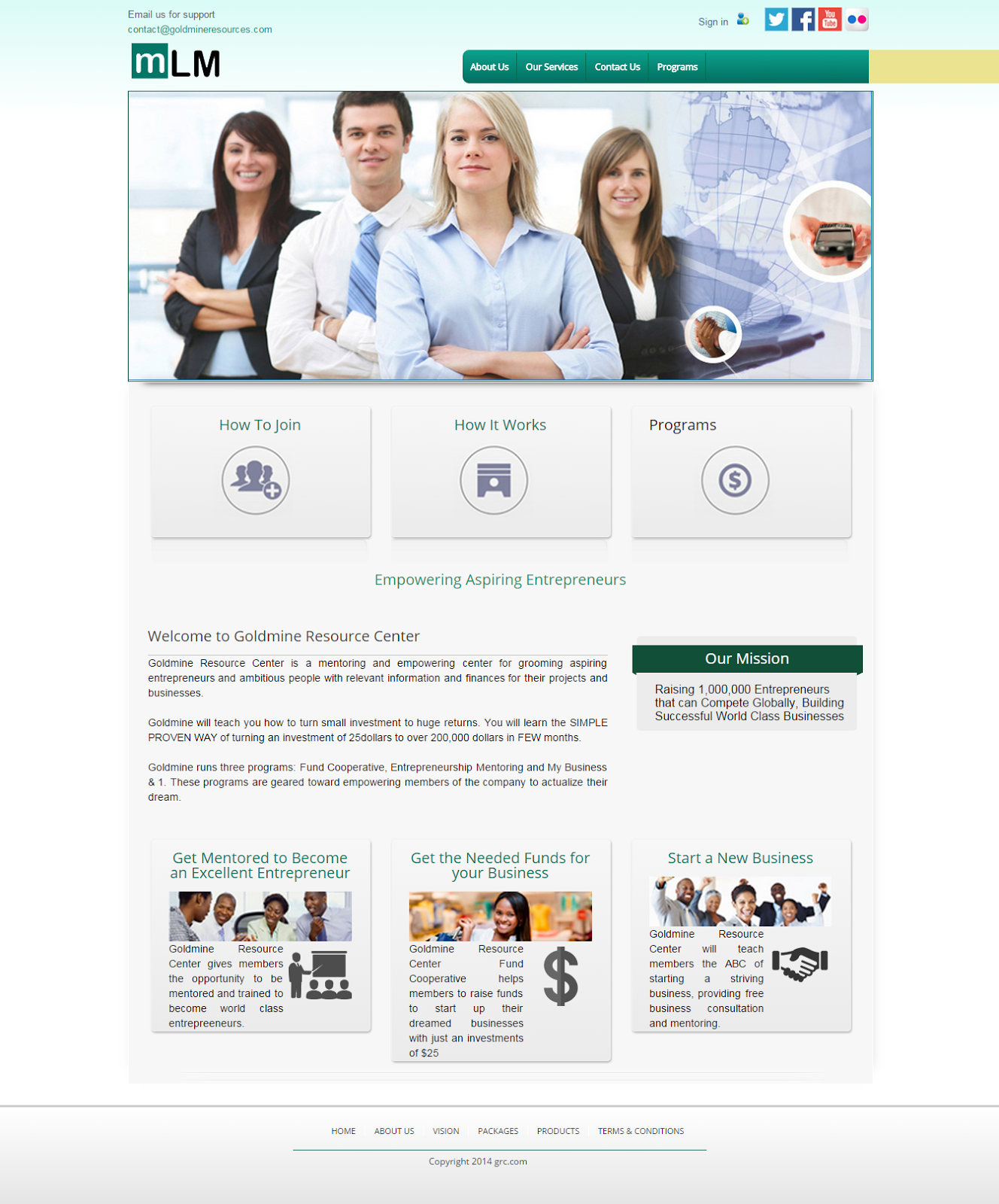The top section of the image features a light green background. Positioned centrally is a green square with a lowercase "m" inside. Adjacent to it, the letters "L" and "M" are displayed in black uppercase text, forming the acronym "MLM." Below this header, there is a rectangle showcasing four individuals. 

On the far left, a woman with dark brown hair smiles warmly. She has her arms crossed and is dressed in a blue shirt under a black jacket. Next to her stands a man with short brown hair, wearing a white collared shirt paired with a blue tie. The third individual is a woman with blonde hair swept to the side; she wears a blue dress shirt and stands with her arms crossed. The fourth person on the far right is another woman with brown hair, also smiling, and dressed in a black and white shirt.

Beneath these individuals, there are three squares labeled "How to Join," "How It Works," and "Programs." Moving down the image, there is a welcoming message that reads "Welcome to Goldmine Resource Center." Adjacent to this, a green rectangle titled "Our Mission" is displayed. Toward the bottom, three more informational squares feature images of people. One square showcases a group of people sitting around a desk, another displays a dollar sign symbol, and the final one depicts a group of people giving a thumbs-up and smiling, promoting the concept of starting a new business.